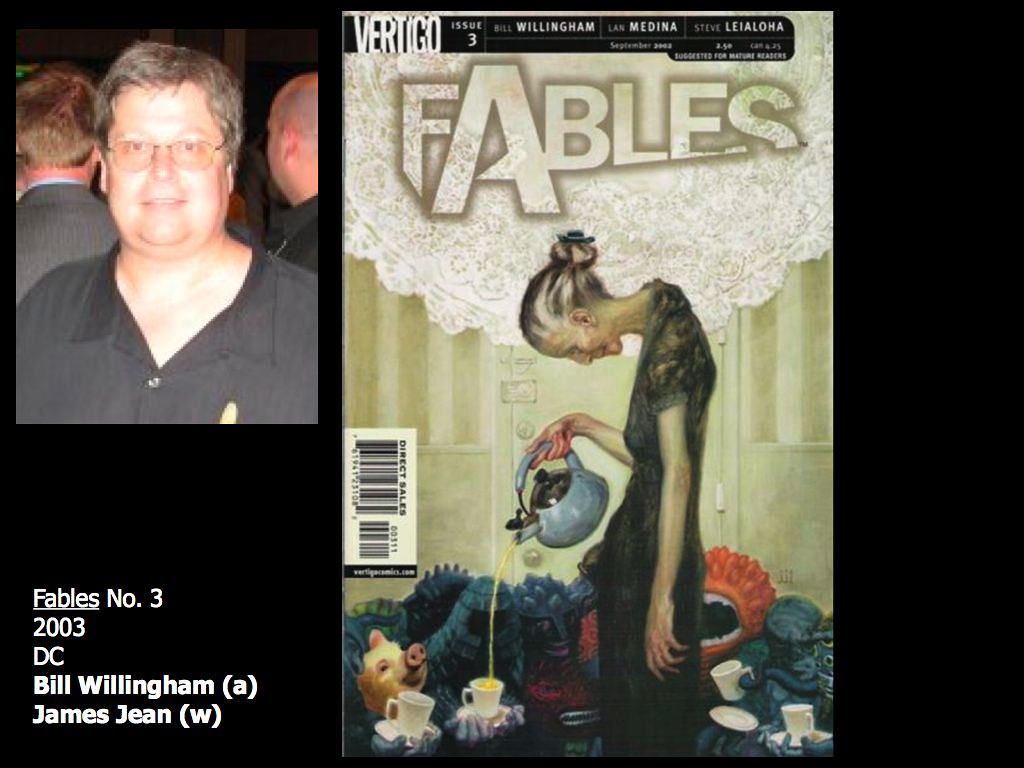This image is the cover of the 2003 DC comic "Fables No. 3," created by Bill Willingham (A.) and James Jean (W.). The cover features a surreal and eerie illustration at the center-right, dominated by a stylized elderly woman hunched over, her neck bent so her head faces directly downwards as she pours tea from a kettle into a cup held by a small figure in blue armor, whose face is obscured by a helmet. The background is populated with ghostly faces and a pig peeking out from behind scattered tea glasses. The top of the image displays a white doily alongside the word "Fables." On the left side, there's a photograph of a man in glasses—one of the authors—looking straight into the camera, with two men positioned behind him. The text above reads, "Vertigo, Issue 3," setting a haunting tone for the cover.